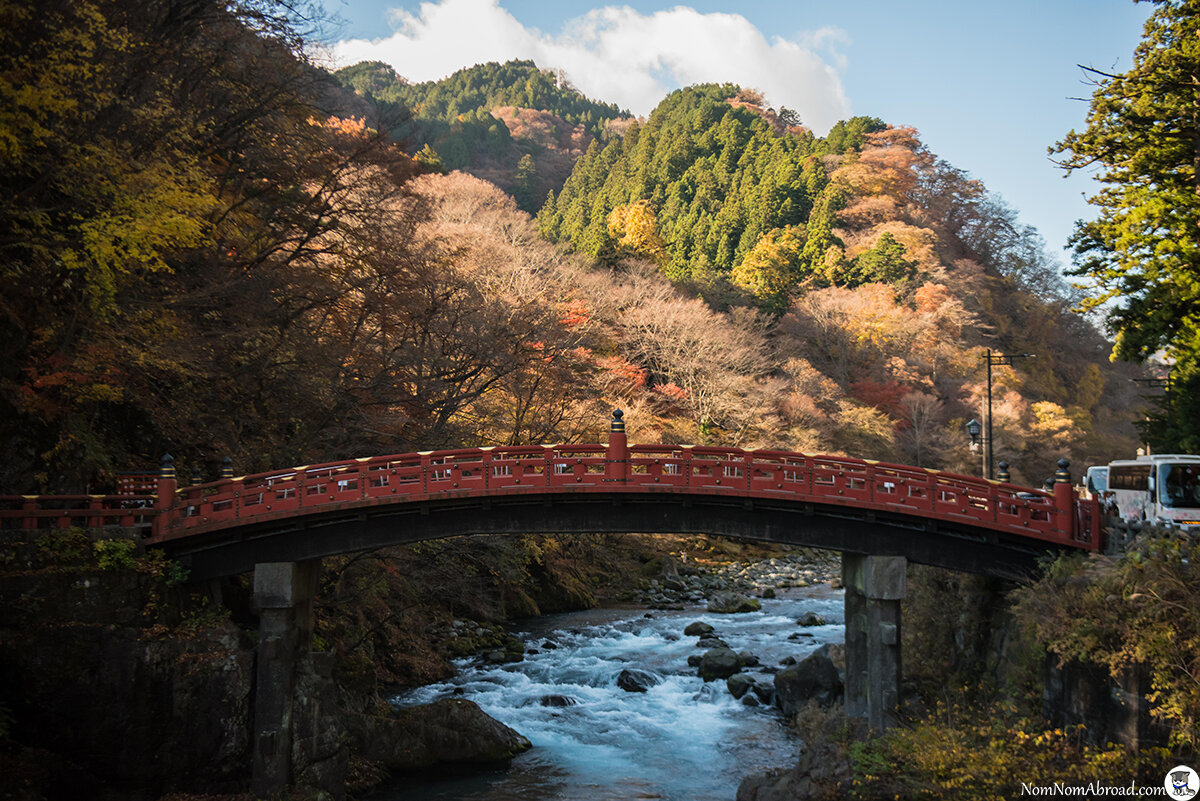This high-quality image captures a beautifully detailed scene of a red, slightly arched wooden bridge, supported by substantial gray columns at either end, stretching over a lively mountain river filled with large rocks and boulders. The bridge, painted a vibrant red and characterized by its low openwork railings, curves gently upward, showcasing an elegant, oriental design. The river below rushes vigorously, creating white water rapids that meander through the rocky banks on either side. In the background, a valley slopes gently upward into a series of hills and mountains adorned with a blend of autumnal foliage. The trees exhibit a rich palette of colors ranging from greens and yellows to reds and browns, interspersed with clusters of evergreens. To the far right of the photograph, near the entrance to the bridge, a white tour bus with smoky windows is visible alongside other parked cars. This picturesque scene of autumnal beauty is framed by the grandeur of nature, offering a stunning view of the changing seasons and the timeless elegance of the bridge.